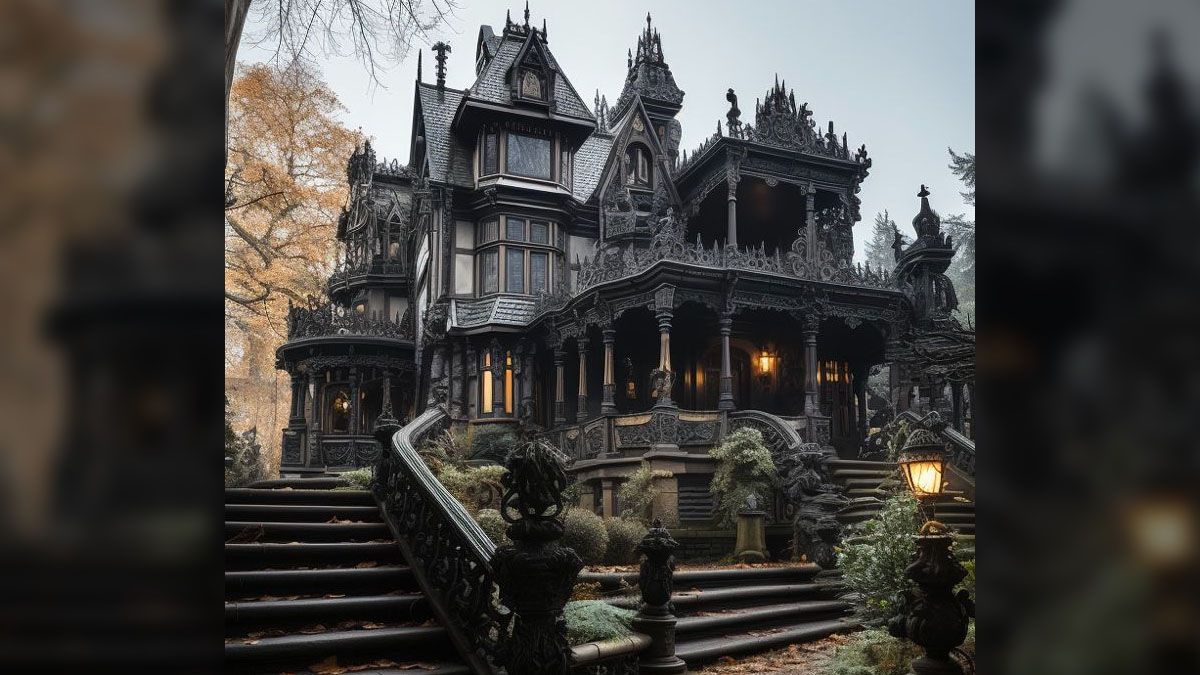The image depicts an imposing, castle-like gothic mansion featuring gray shingles, black accents, and large, intricate steeples and window dressings akin to a medieval castle. Central to its grand architecture are multiple stories marked by massive stone pillars that frame the structure. The mansion boasts several entrance points accessed by expansive stone staircases located at the left, right, and center. Stone statues adorn the right side of the home, adding to its gothic allure.

Illuminating the mansion are numerous lights, some set on pedestals and others shining from various windows, creating a warm glow against the predominantly gray exterior. Amidst the intricate design are patches of greenery, with multiple plants in various shades of green placed in a central courtyard and surrounding areas. The background showcases tall trees, with evergreens on the right and deciduous trees with fall-colored leaves on the left, all under a clear blue sky.

The artwork gives a slightly blurred, painterly effect, suggesting that the image may be an artist's rendition rather than a photograph. Despite this artistic blur, the mansion remains the focal point with its sharp, towering edges and cathedral-like elements.